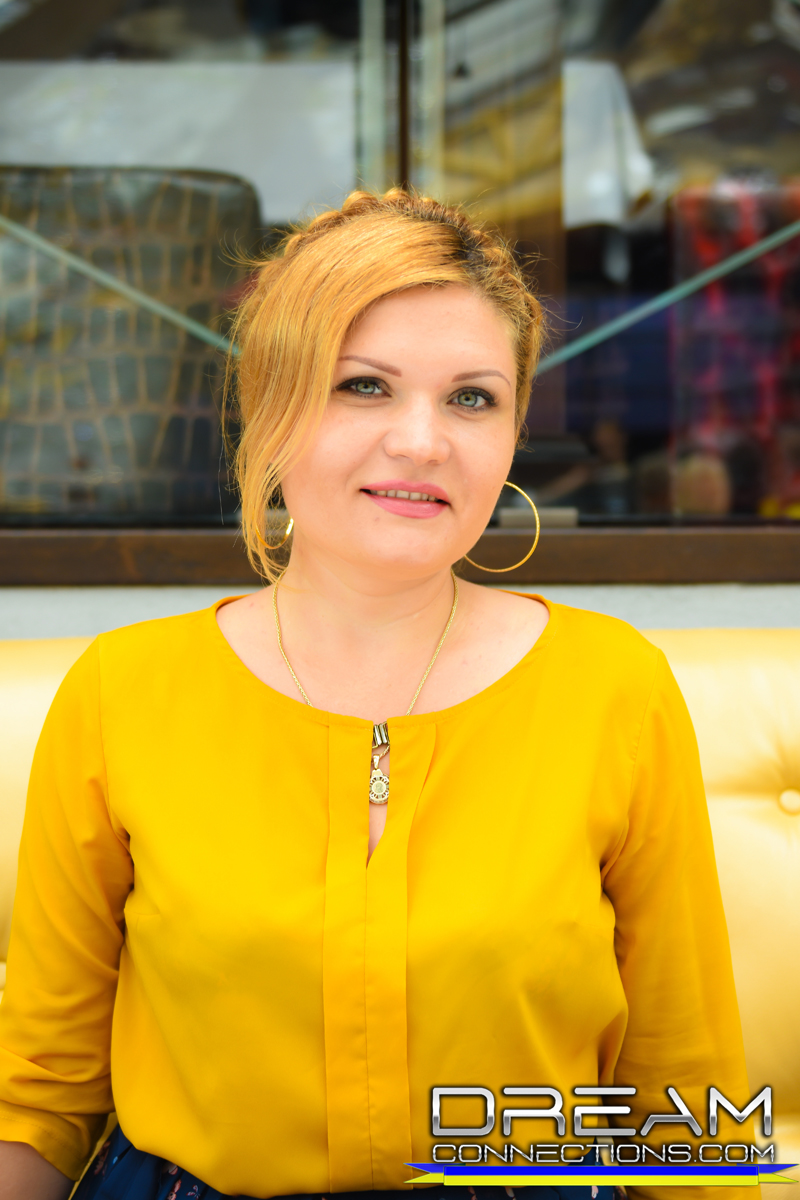In the center of the image, there is a young woman with yellowish blonde hair that has dark roots, styled in a braid going from front to back. She is looking directly at the camera with a pleasant expression. She is wearing a long-sleeved, golden button-down shirt and a gold-colored necklace with something silver hanging from it, partly obscured by the shirt's opening. The woman appears to be in her mid to late twenties or early thirties.

Behind her, there is a window or possibly a display case with a wooden frame and glass, showing reflections. Inside, on the left, there is a native African drum and other indistinct items on the right. The background scene includes a picture with brown, crosshatched lines and teal green diagonals as well as some reddish and gold color elements.

The image, predominantly featuring colors like brown, black, tan, yellow, blue, and red, looks like it could be an introductory photograph for a model or participant, possibly for a dating website. In the bottom right corner, the text "dreamconnections.com" is visible, with "Dream" stylized in blue and "Connections.com" in capital letters with a blue stripe underneath.